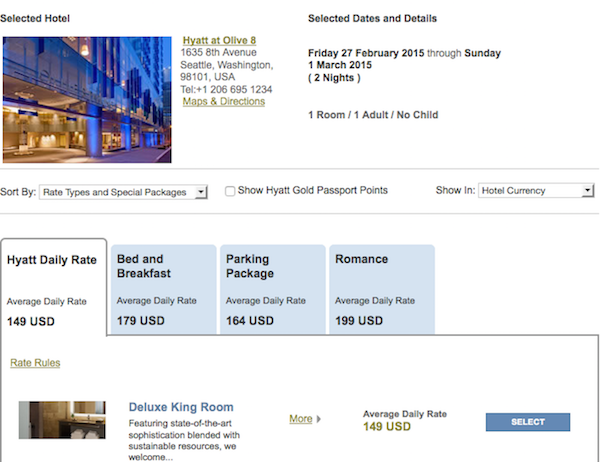Screenshot of a travel or hotel booking website showcasing details for a selected hotel, the Hyatt at Olive 8. 

In the upper left-hand corner, the name of the hotel is prominently displayed alongside its address, with a link provided for maps and directions. To the left of this section is a nighttime image of the hotel exterior.

To the right, the selected dates and details are clearly outlined: Friday, 27 February 2015 to Sunday, 1 March 2015, for a two-night stay. The reservation is specified for one room accommodating one adult with no children. 

The website background is white with various sections. Just below the main details, a horizontal strip features sorting options through a drop-down menu, along with checkboxes for displaying Hyatt Gold Passport points and pricing in the hotel's local currency.

Below this, four room packages are available: Hyatt Daily Rate Room, Bed and Breakfast, Parking Package, and Romance Package. The selected package is the Hyatt Daily Rate. The average daily rate is listed at $149, and the chosen room type is the Deluxe King Room, illustrated by a small image to the left.

The room description highlights "state-of-the-art sophistication blended with sustainable resources," and includes a "More" link button for additional details. The daily rate is reiterated at $149, with a blue "Select" button to the right. The other room package tabs remain unselected, displayed in a white and blue color scheme with varying prices.